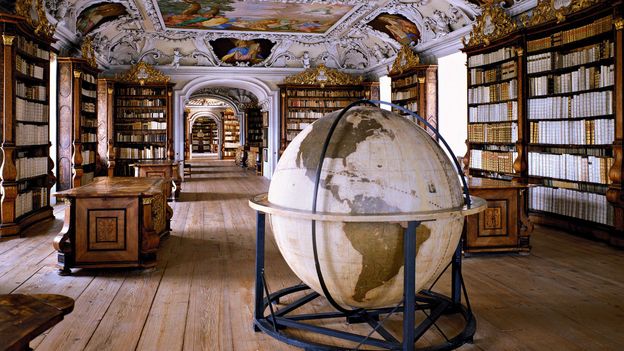The image captures a grand, Renaissance-style library with an air of opulence and historical charm. Dominating the foreground is a massive globe featuring continents in brown and oceans in hues ranging from white to beige, all supported by an elaborate black wrought iron stand. The library's ceiling is adorned with vibrant, intricate paintings in greens, blues, and yellows, framed by ornate moldings that enhance its European elegance.

The room is expansive, with walls lined by towering bookshelves, most of which house books with white spines, though variations in orange and brown are also visible. There are two stately wooden desks positioned symmetrically on either side of the globe, and the entire scene is set against a backdrop of rich wooden floors.

Adding to the grandeur, a large archway with a wooden door trim at the back of the room reveals additional corridors filled with more books. The floor-to-ceiling windows flood the space with natural light, highlighting the detailed gold tops and wood bases of the bookshelves. Overall, this library exudes an old-world sophistication, offering a glimpse into a seemingly endless repository of knowledge.